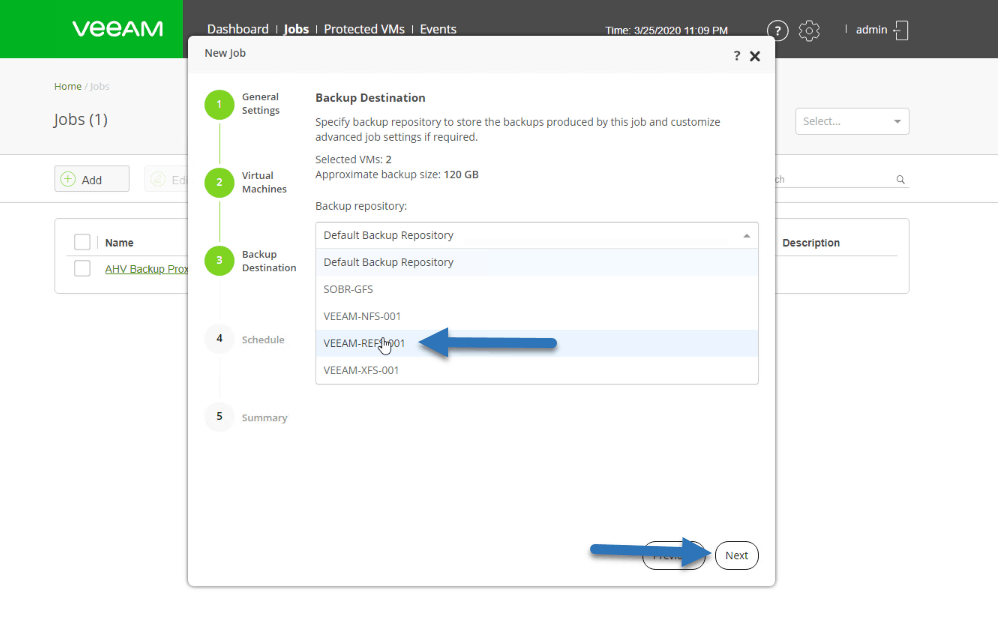The image depicts a screenshot of the Veeam Backup & Replication interface. In the top left corner, there's a green banner displaying the white text "veeam" with "vee" in lowercase and "AM" in uppercase. Below that banner, on the left side of the screen, you see a navigation path "Home / Jobs," followed by "Jobs (1)" in parentheses, alongside an add button.

Beneath the navigation path, there's a partially obscured field labeled "Name," with the text "AHV Backup Proxy," which is blocked by a pop-up window.

The pop-up window is titled "New Job." On the left side of this window, there is a vertical, sequential list consisting of several steps. These steps are: 
1. "General Settings" marked with a green '1'
2. "Virtual Machines" marked with a green '2'
3. "Backup Destination" marked with a green '3'
4. "Schedule," which appears grayed out
5. "Summary," also grayed out

On the right side of the window, the "Backup Destination" step is active. It contains instructions to "Specify backup repository to store the backups produced by this job and customize advanced job settings if required." Below, there's a section titled "Selected VMs," indicating an approximate backup size of 120 gigabytes.

A repository dropdown chart shows various storage options, including "SOBR GFS" and "VEEAM NFS 001" among others. A blue arrow is pointing towards the second to last repository option.

In the bottom right corner of the pop-up window, there's another blue arrow pointing to a "Next" button.